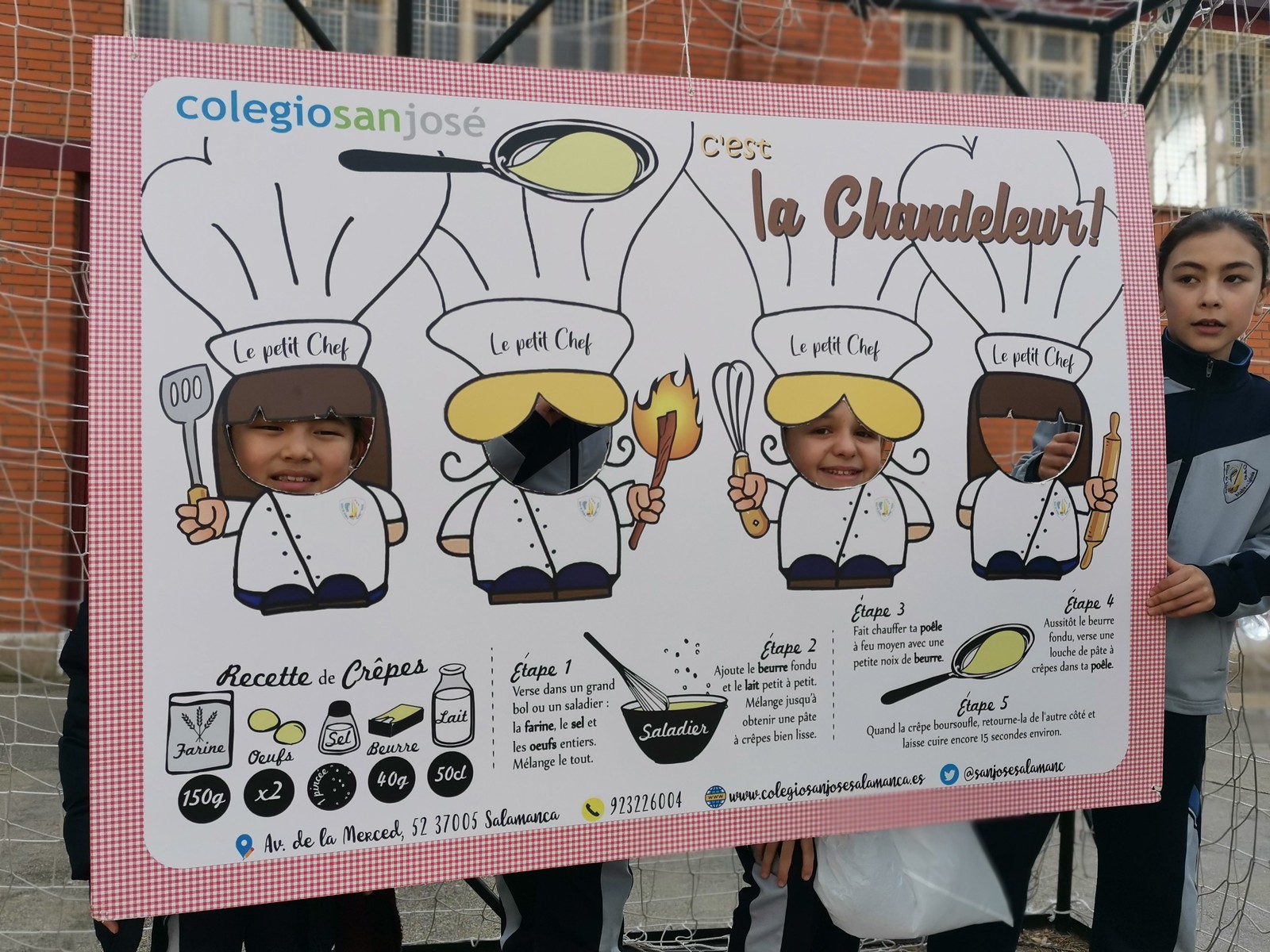In the image, a large poster board showcases four charming animated drawings of chefs, complete with traditional toques and miniature bodies. The faces of these chefs have been cut out to create an interactive photo opportunity. Two individuals are seen standing behind the board, joyfully poking their faces through the cutouts of two of the chef illustrations. Off to the right side, a girl wearing a jacket holds onto the poster, adding to the playful scene. Below the chef illustrations, the bottom part of the poster features detailed text written in French, clearly presenting a recipe for crepes. The recipe includes a list of ingredients with their measurements and outlines five steps to follow.